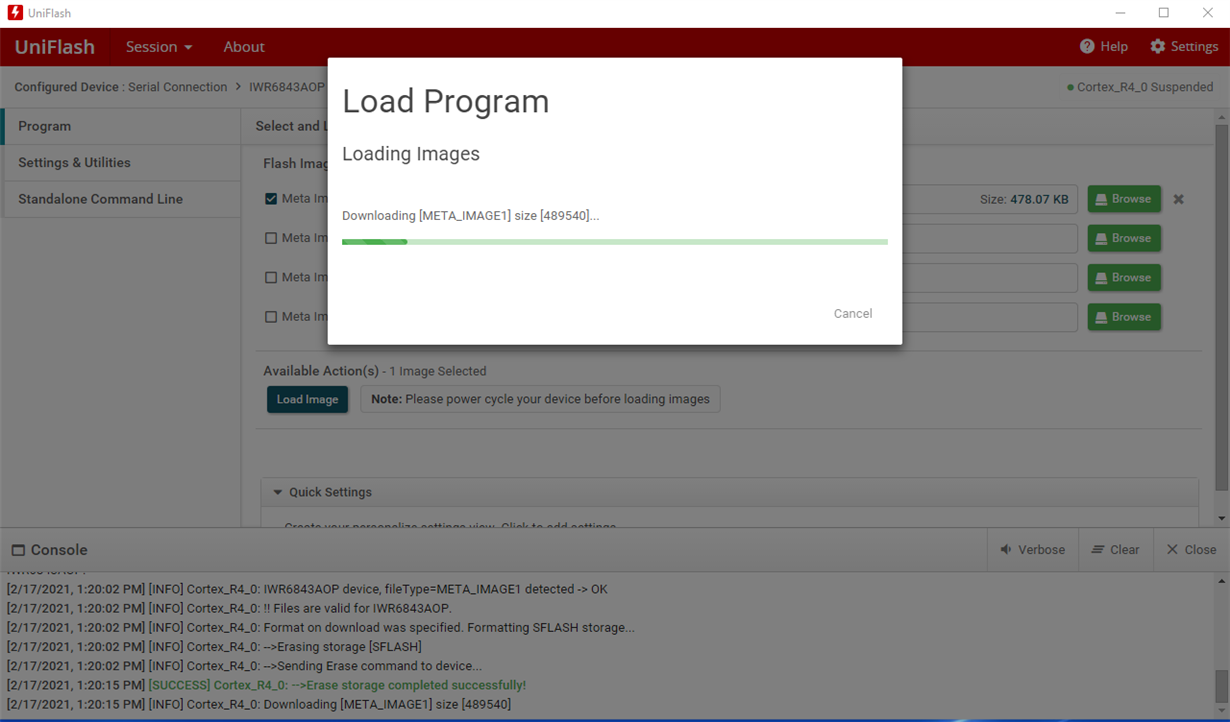Caption: 

The image depicts a website titled "UniFlash," which has a gray overlay covering its interface. Central to the screen is a white dialog box with the bold title "Loading Program." Below this title, text reads "Loading images... Downloading [M_meta_image_1] size [4895040]..." followed by an ellipsis. A progress bar spans across the dialog box, predominantly light green with a hint of dark green signifying progression. In the bottom right corner of the dialog box, there is a "Cancel" button.

Beneath the dialog box, the partially visible website features a red top strip with the label "UniFlash." This strip includes a dropdown menu labeled "Season" and links for "About," "Help," and "Settings" on the right side. Below the top strip, a left-justified vertical menu lists options: "Configure Device," "Program Settings," "Utilities," and "Standalone Command Line."

The dialog box obscures portions of the interface, cutting off some of the menu text. Visible yet truncated labels include "Select," "Flash," and "Meta," indicating interactive elements on the webpage. To the right, partially hidden by the dialog box, are four green "Browse" buttons arranged vertically.